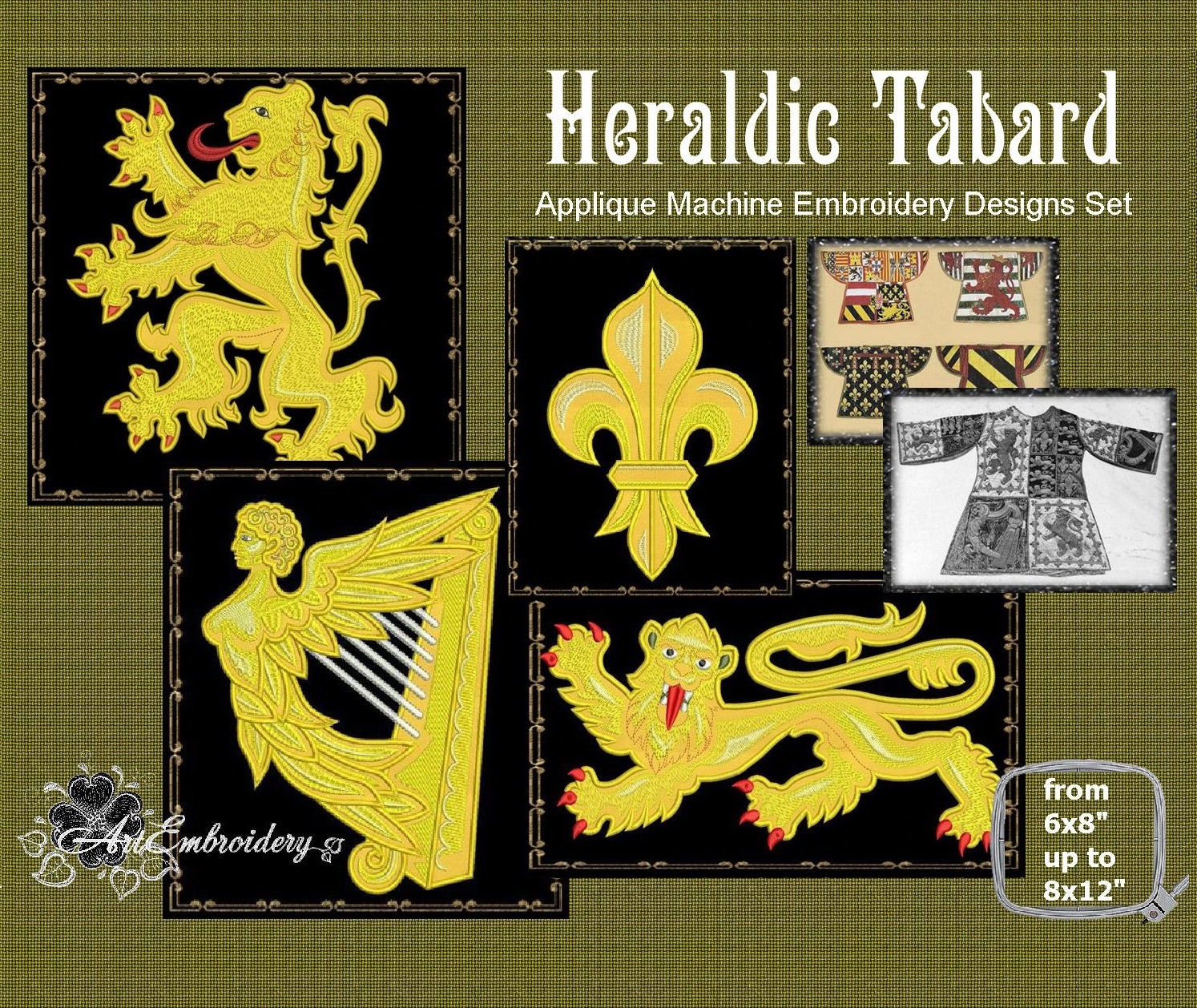The graphic features a display with a light brown or olive green background, prominently showcasing embroidery designs. In the upper right-hand corner, it reads "Heraldic Tabard Appliqué Machine Embroidery Designs Set" in bold, medieval-style white text. The bottom left corner is labeled "Art Embroidery," while the bottom right mentions the sizes available: "From 6 x 8 inches up to 8 x 12 inches." Central to the graphic are several intricate embroidery designs. These include multiple poses of a regal lion, a gold harp adorned with an angel on one side, and a classic fleur-de-lis, all rendered in vibrant, colorful patterns. Some designs appear to be applied to textile samples, hinting at their practical applications.